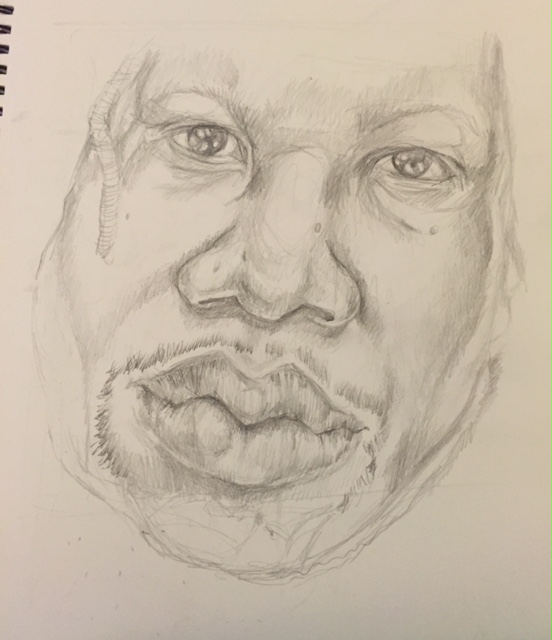This is a slightly vertically-oriented pencil sketch of a man's face on dark cream-colored paper. The subject appears to be an African American man in his 50s, characterized by his goatee that frames a thin mustache and continues down around his chin. He has thick lips and a wide nose. The top part of the sketch fades out, making it difficult to discern his hairstyle. The lines around his cheeks are somewhat indistinct, particularly on the left side from the viewer's perspective. A dreadlock or similar feature cascades down along his right temple. In the upper left corner, a small part of the spiral binding of the notebook is visible, enhancing the authentic, sketchbook feel of the artwork.